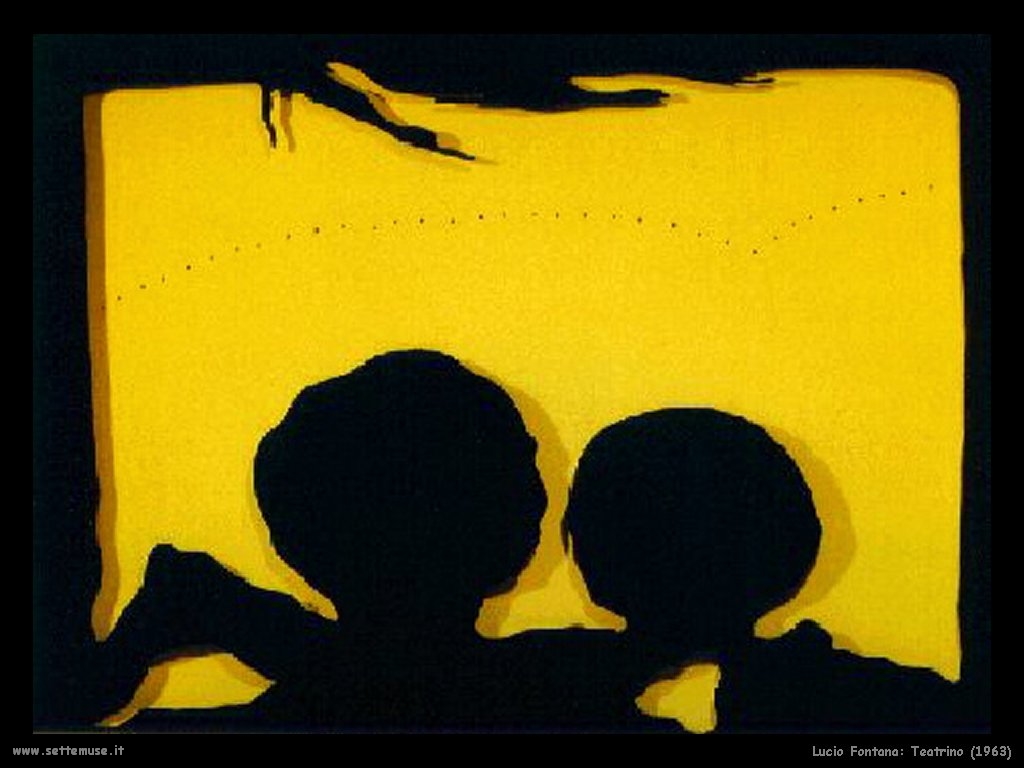In this striking and unique artwork, created by Lucio Fontana in 1963, the scene is dominated by the silhouettes of a man and a woman in embrace, rendered entirely in black against a vibrant, bumblebee yellow background. Centered towards the bottom of the image, their outlines are distinct yet open to interpretation, giving a sense of intimacy and connection. The yellow backdrop, reminiscent of a television screen, features a scattering of tiny black dots running horizontally, adding texture and depth to the scene. Branch-like black lines hang down from the top, partially intruding into the yellow space. Encircling the art is a bold black border, which intensifies the contrast and frames the composition compellingly. The bottom left corner bears the website www.setmuse.it, while the right corner is inscribed with "Lucio Fontana: Titrino 1963," grounding the abstract imagery in historical context.